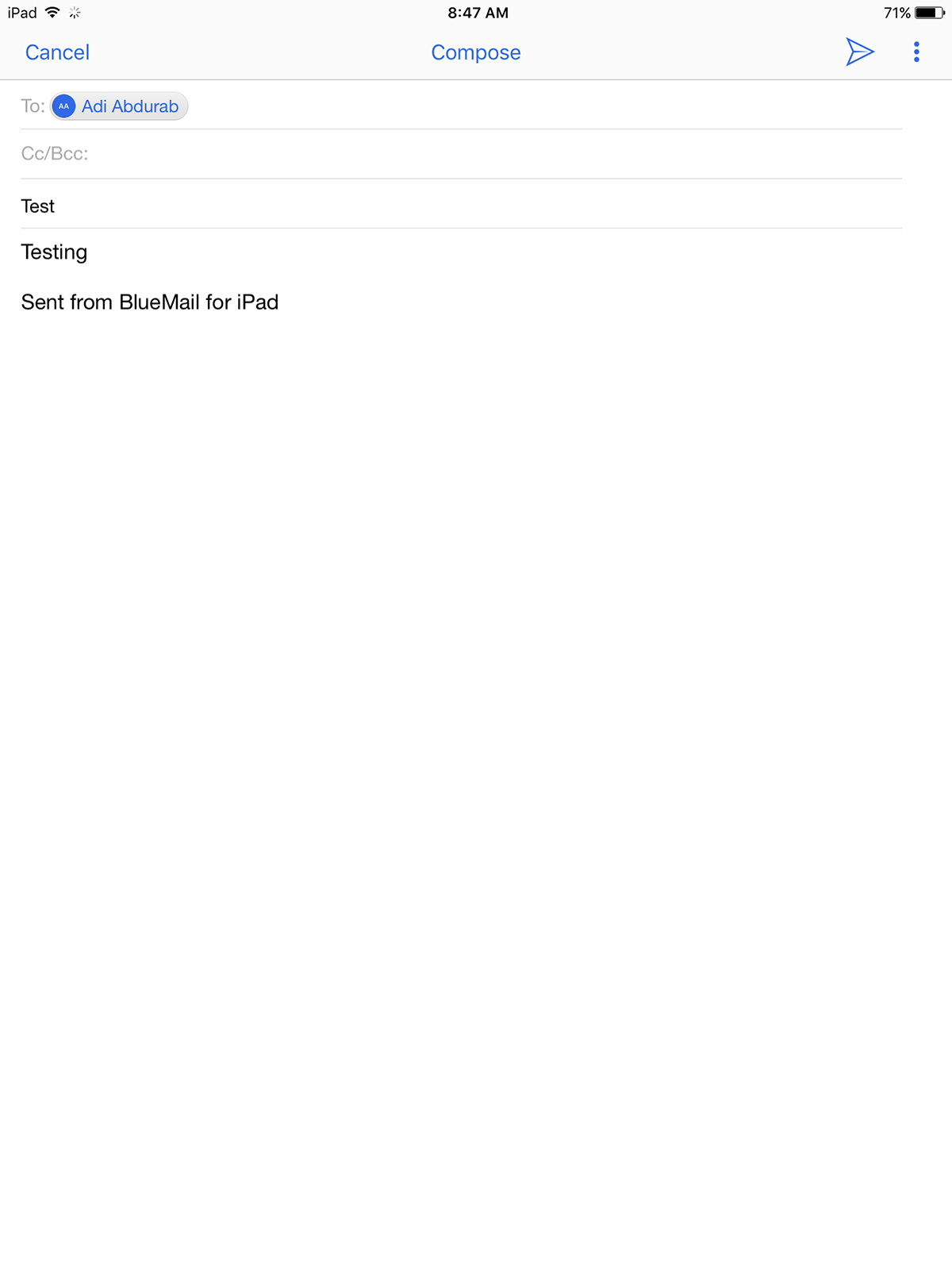Screenshot of an iPad interface with a white background. In the upper left corner, the word "iPad" is displayed next to an internet connection icon and a sunburst-like settings icon. The center of the screen shows the current time as 8:47 AM. On the upper right, the battery level indicates 71% charge.

Below this, there is a navigation bar with the word "Cancel" in blue on the left, "Compose" in blue in the middle, and a blue right-pointing triangle followed by three blue dots on the right. 

The main body of the screen displays:
- "2TO:" followed by a gray oval, a gray rectangle, and a blue circle with two 'A's inside it, next to the name "ADI ABDURAB."
- Below this, "CC/BCC:" in light gray.
- Under this section, a line of text reads "test" in dark black.
- Beneath that, another line says "testing" in dark black.
- Finally, at the bottom, the text "Sent from Blue Mail for iPad" appears in black.